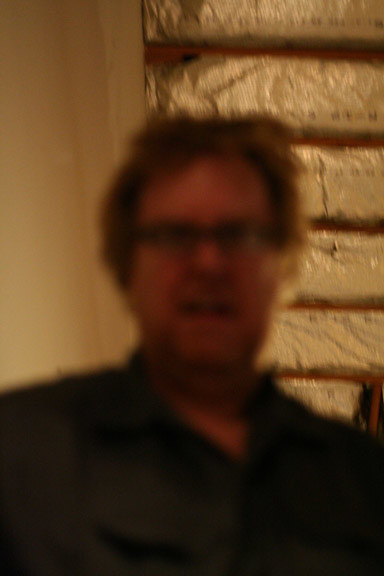A blurry and grainy photograph captures the surprised or angry expression of a white man with medium-length curly hair and an unkempt beard, suggesting he is in his late 40s. He is wearing glasses and a black collared shirt. The poor image quality indicates it may have been taken from a distance and heavily zoomed in, or possibly captured while in motion.